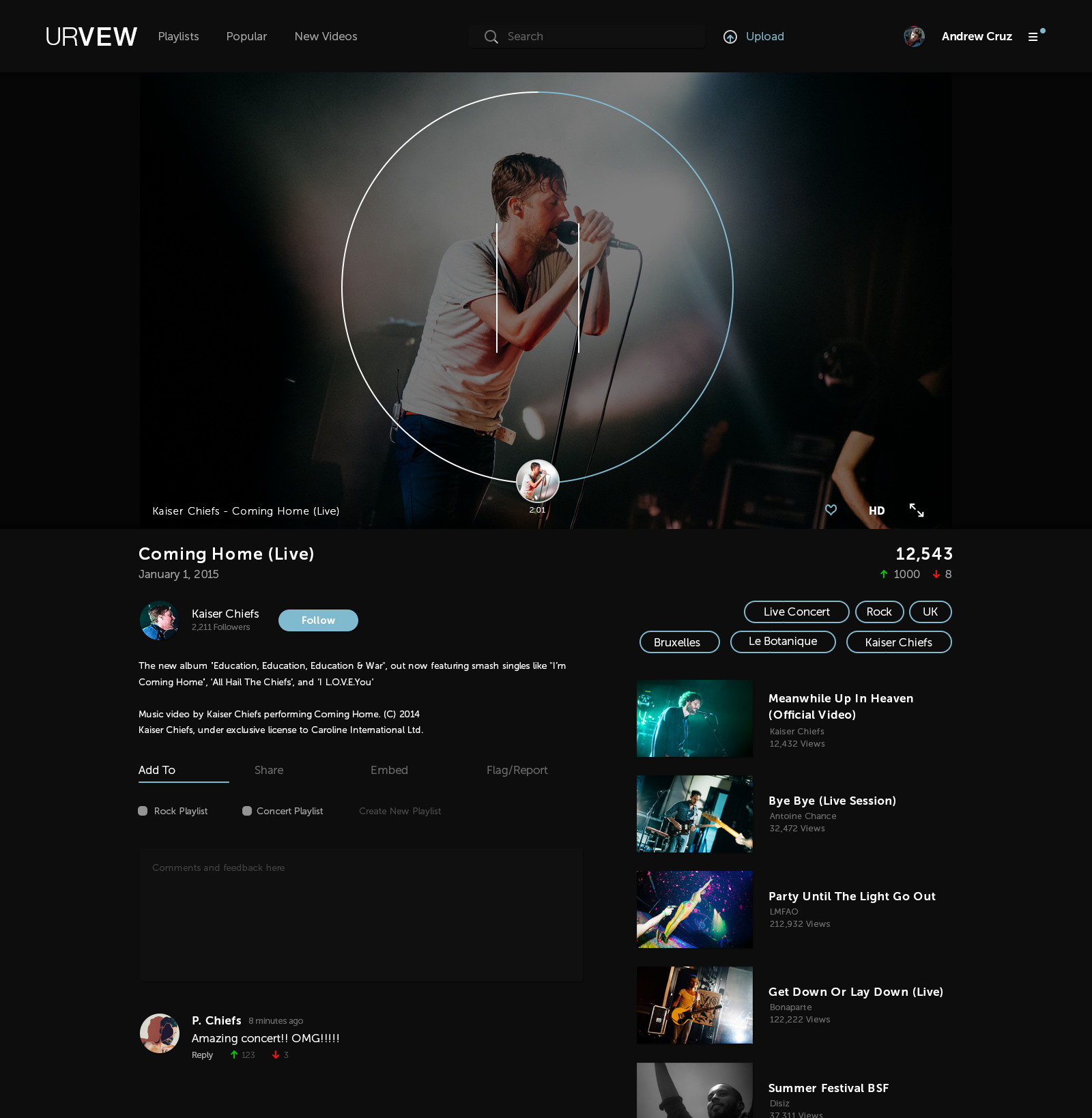This image is a screenshot of a video streaming website named "You are", stylized as "You are VW". At the top left, the website’s name is prominently displayed. Moving from left to right across the top of the page, there are several tabs labeled "Playlists", "Popular", and "New Videos". Further to the right, there's a "Search" bar followed by an "Upload" button. In the top right corner, the name "Andrew Cruz" is displayed next to an icon resembling a hammer, which features a small green dot, indicative of a notification.

Centrally displayed on the page is a live video feed of a man who appears very sweaty, with wet hair and passionately singing into a microphone, suggesting a high-energy performance. The video is part of a concert titled "Coming Home", streamed live on January 1, 2015. The event is currently being viewed by 12,543 people, implying the platform’s capability to support large, virtual concert audiences.